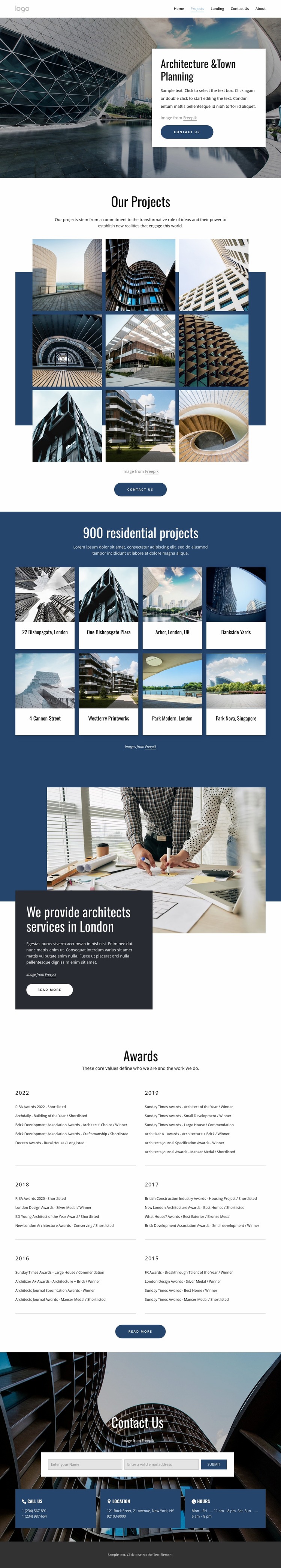The image showcases a composite of four different web pages, each shrunken to a size that makes discerning detailed information quite challenging. The topmost section features a small rectangular image, possibly depicting the front of a car. Within this image, there is a white rectangle containing text, the first word of which might be "architecture," followed by unreadable words that could pertain to planning.

Directly below this is another rectangular section titled "Our Projects," featuring six diminutive images. The picture on the far left appears to be a stadium, though the small size makes it difficult to confirm. Among these images is one that resembles a high-rise building with numerous windows.

The third section below contains a square with the text "900 residential projects" printed in white. Beneath this text, there are eight tiny images, which seem to depict different mountain landscapes, though the small size again limits clarity and detail.